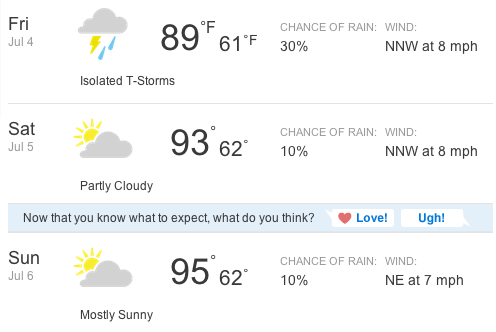This image showcases a detailed five-day weather forecast from a digital platform, presented in landscape orientation against a white background. The frame has minimal visual boundaries, with only a slim gray line tracing the left edge. The forecast days are organized horizontally with clear dividers.

1. **Friday, July 4th**:
   - **Weather Icon**: A cloud with a lightning bolt and two raindrops.
   - **Description**: Isolated thunderstorms.
   - **Temperature**: High of 89°F, Low of 61°F.
   - **Precipitation Probability**: 30% chance of rain.
   - **Wind**: North-northwest at 8 mph.

2. **Saturday, July 5th**:
   - **Weather Icon**: Partly cloudy.
   - **Temperature**: High of 93°F, Low of 62°F.
   - **Precipitation Probability**: 10% chance of rain.
   - **Wind**: North-northwest at 8 mph.

3. **Information Banner**:
   - The banner declares, "Now you know what to expect. What do you think?" with clickable options to rate the forecast as "love" or "uh," inset within a blue bar.

4. **Sunday, July 6th**:
   - **Weather Icon**: Mostly sunny.
   - **Temperature**: High of 95°F, Low of 62°F.
   - **Precipitation Probability**: 8% chance of rain.
   - **Wind**: Northeast at 7 mph.

Each day’s forecast is visually separated by horizontal lines, enhancing clarity and organization.